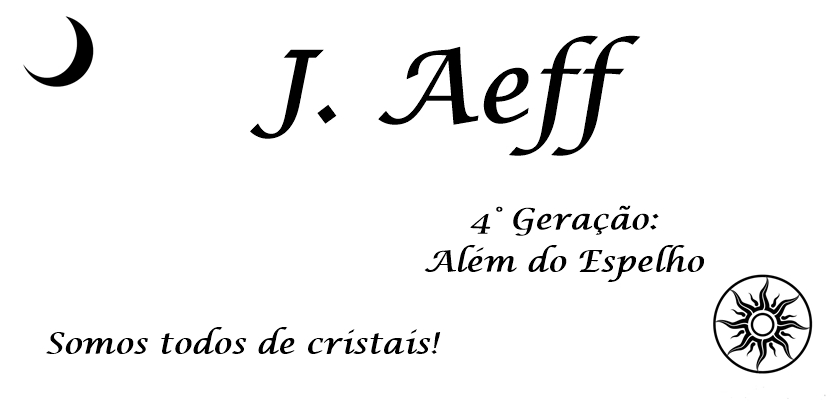The image features a plain white background with black italic text centered across it. At the top, in large bold and italicized letters, is the text "J. A-E-F-F" accompanied by a crescent moon in the upper left corner, with the open end facing the corner. Below this, in smaller italic font, is the phrase "4º Geração: Além do Espelho." Along the bottom, in the same italic font, is the phrase "Somos Todos de Cristais!" In the lower right-hand corner, there's a circular emblem with a detailed mandala pattern resembling a sunburst, characterized by wavy rays emanating from a central circle.